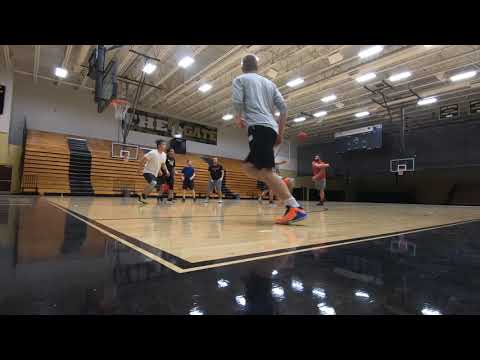The indoor basketball court image displays a dynamic basketball game in progress, captured from a floor-level viewpoint. The sleek, light wooden court floor, reflecting the bright ceiling lights, dominates the lower half of the image, bordered by black sections. The players, six to seven men, are dressed in various casual outfits without team uniforms, making it hard to distinguish between teams. Central to the scene, a player in red is poised to throw the ball to another player in gray, who is turned away from the camera. In the background, the folded-up bleachers line the wall beneath a sign reading "The Gate." Multiple basketball hoops and backboards are visible, two on the left and one on the right. The court is brightly lit, with the open metal structure of the ceiling filled with lights that cast reflections on the pristine floor.